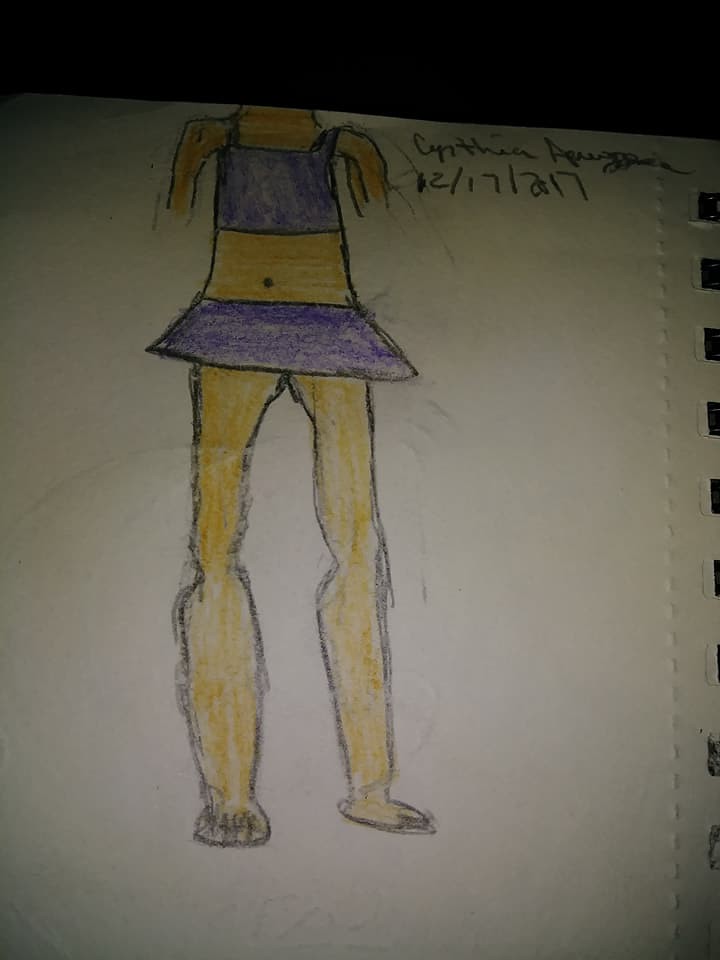This is a detailed drawing, likely by a young artist, of a headless girl depicted from the neck down, created using both pencil and crayon on a piece of white paper. The figure is dressed in a purple halter top that ends just above the belly button, paired with a short, matching purple skirt. The girl's arms are only partially drawn, stopping at the upper arms and leaving the forearms and hands unfinished. Her body is colored in a darker peach or tan shade, suggesting an effort to depict a specific skin tone. The legs are long and notably disproportionate, featuring very large calves and small, somewhat awkwardly positioned feet. One foot is turned sideways, adding an interesting detail to the drawing. The image has visible pencil outlines, with multiple attempts and visible corrections marked by scratch-outs. Above the figure, the name "Cynthia" is written, followed by an incomplete last name, and a date "12-17-2017."